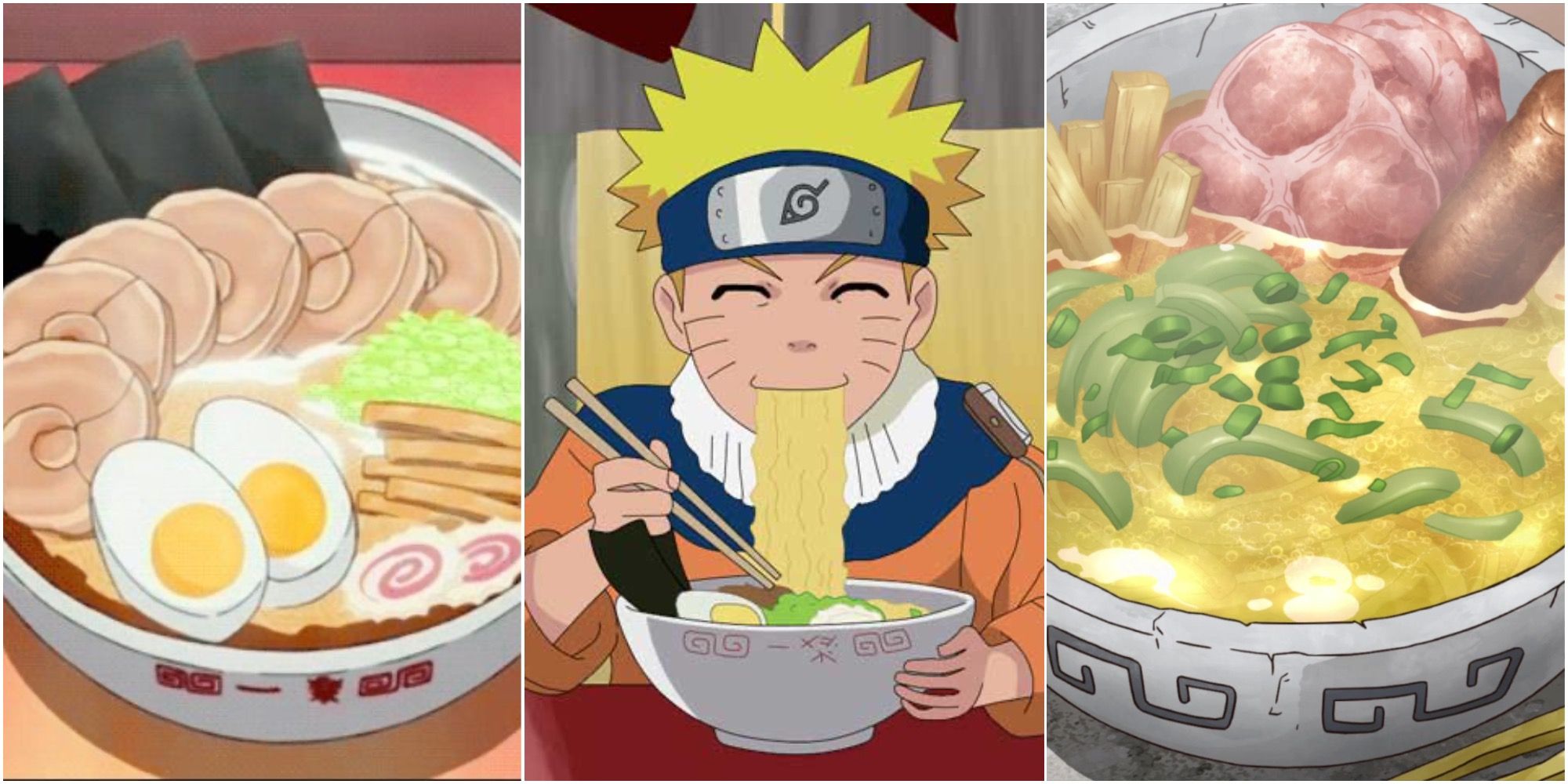The image consists of three vertically divided, hand-drawn illustrations related to oriental food, specifically various types of ramen. The left panel portrays a white bowl filled with ramen, featuring two halves of a hard-boiled egg, several pieces of meat, black seaweed strips, yellow Uzumaki spirals, green lettuce, and what appears to be non-fried potato-like sticks. Oriental writing is visible on the bowl. The center panel showcases a young, manga-anime style character, identified as Naruto, with spiky blonde hair. He wears a blue headband with a silver plaque displaying a pyramid or chili pepper symbol, and an orange tunic with a white stand-up collar. Naruto is smiling with closed eyes, slurping noodles from a large white bowl using chopsticks. The right panel presents another white bowl of ramen with a yellowish broth, chopped scallions, pink meat, a brown stick-like item, and various unidentifiable long vegetables. The entire illustration is detailed and colorful, with a distinct manga anime style throughout, encapsulating the essence of oriental cuisine.